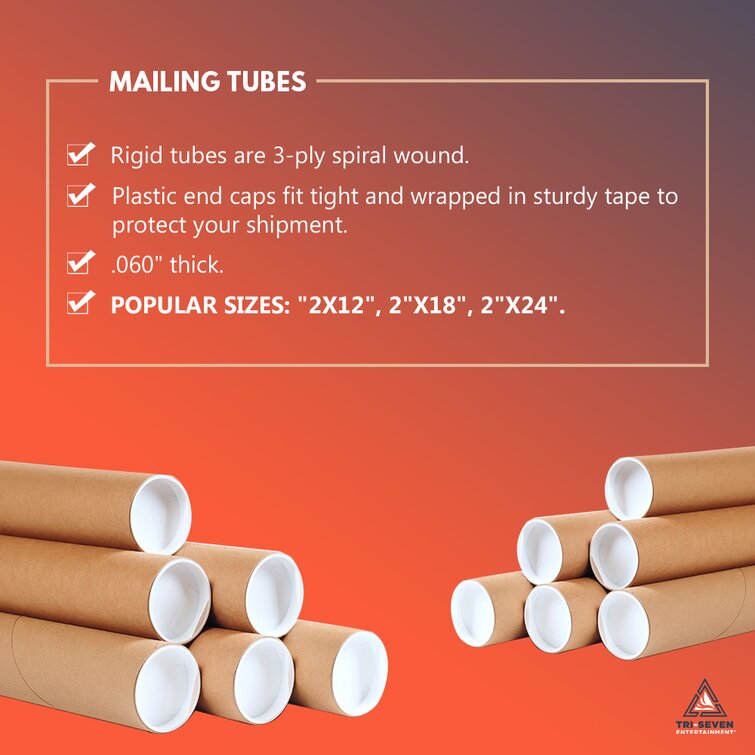This detailed advertisement features mailing tubes with a vibrant orange background. At the top, white text clearly states "Mailing Tubes," accompanied by an extensive checklist detailing the product features: "Rigid tubes are three-ply spiral wound, 0.060 inches thick, plastic end caps fit tightly and are wrapped in sturdy tape to protect your shipment." The advertisement highlights popular sizes: 2x12, 2x18, and 2x24 inches. Below the checklist, two photographs display the mailing tubes, each brown with white caps and arranged in two stacks of six. In the lower right corner, a logo featuring a triangle and the company name, "Try 7," signifies the brand. Sharp edges frame the image, enhancing its bold, clear design.